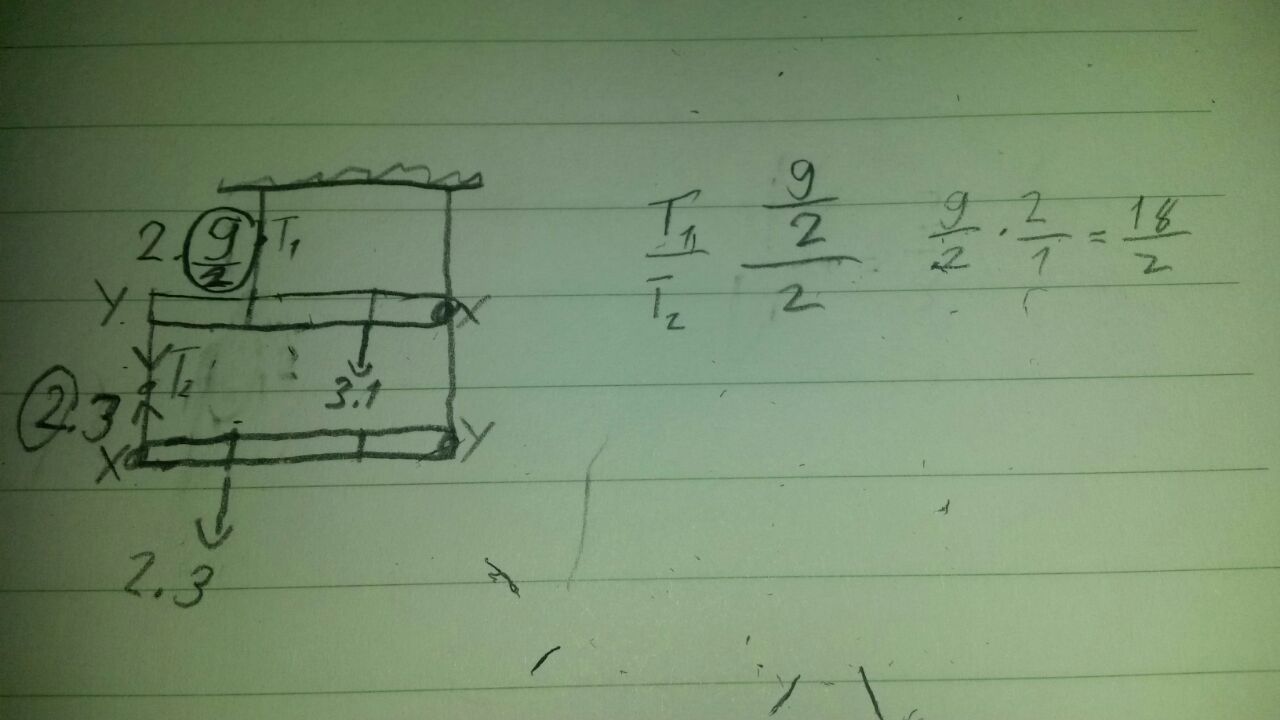The image showcases a white sheet of paper with gray horizontal lines. The paper, oriented in a landscape format, appears to have been used for some mathematical calculations and sketches, all roughly drawn with a pencil. 

On the right side of the page, a series of mathematical equations are visible, beginning with "T subscript 1 over T subscript 2." Adjacent to this, a fraction "9 over 2" is notated, followed by its simplification process demonstrated as "9 over 2 times 2 over 1 equals 18 over 2."

Towards the left side, two rectangular boxes are sketched, with the smaller box positioned above and slightly to the right of the larger one, aligning at their right edges. Within these boxes, variables "X," "Y," and "Y3" are indicated. The top box has a circle around the fraction "9 over 2," while the bottom box contains a circle around the number "2" next to "3," with an arrow pointing down towards "2.3."

The surface of the paper is dotted with scattered spots of graphite, adding to the sketch's informal and somewhat cluttered appearance.